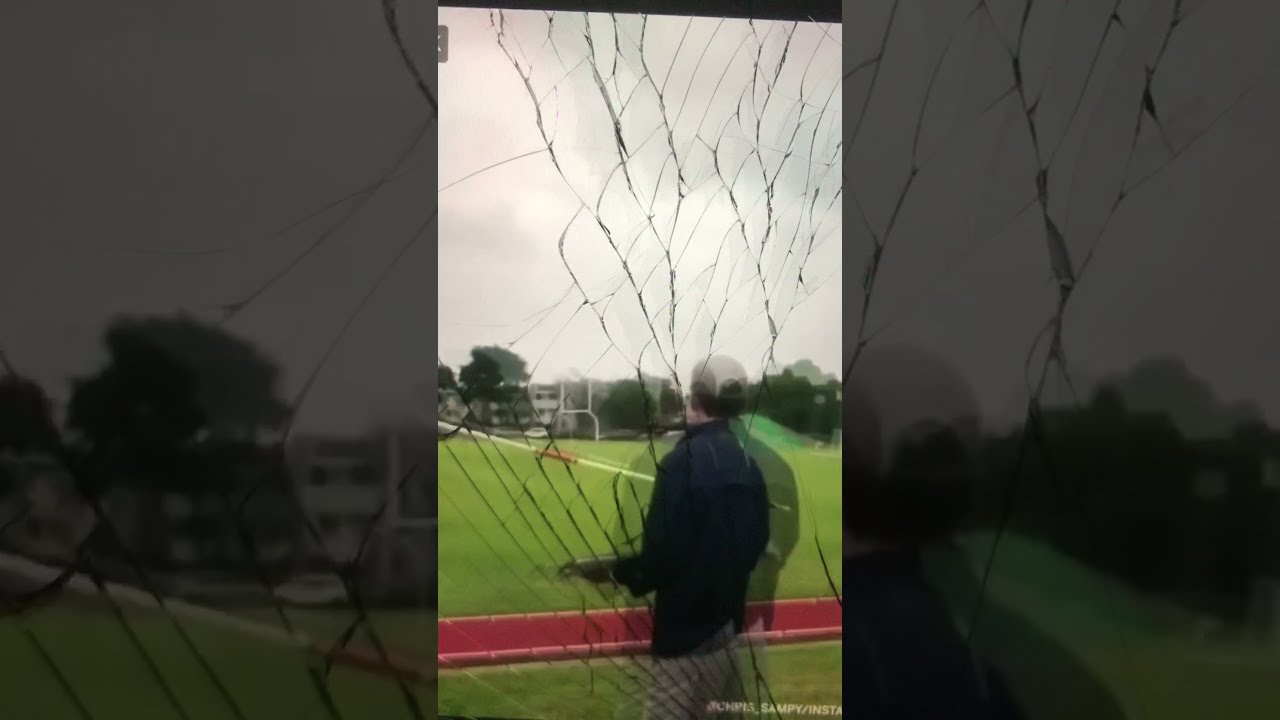A blurred image of a person standing in front of a net shows multiple shifting moments, affecting both the individual and their background. The person, clad in a dark jacket, light-colored pants, and a light hat, faces away from the camera. Behind them, a red track, which remains unduplicated and framed by white bars, extends horizontally. Green grass dominates the field, framed by the track. In the distance, a goalpost appears in front of trees, with multi-story white buildings discernible further back. The sky, occupying the upper half of the image, is a mix of white and blue. The image includes the appearance of cracked glass overlaying it, suggesting a photo taken of a phone screen. This cracked glass creates numerous fractures, obscuring much of the view. Below this, text partially reads "S-A-M-P-Y-I-N-S-T-A" while a more legible watermark at the bottom right corner states "@chris_sampy/insta”. Wide, grayed-out borders on the left and right sides, which are enlarged details from the central image, frame the central, narrow portion of the image.